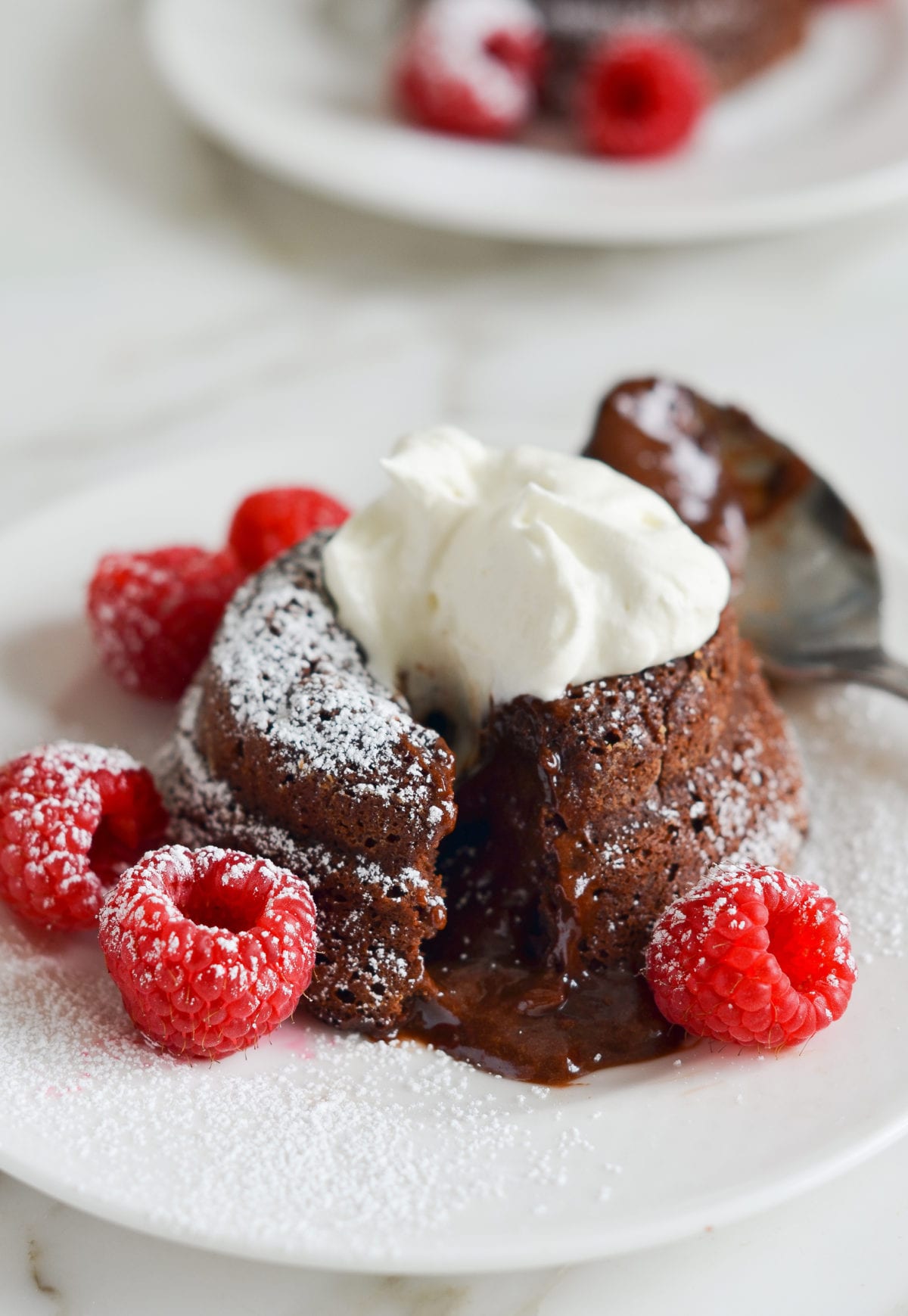The close-up photograph showcases an indulgent chocolate lava cake, its round, cake-like structure partially opened to reveal a rich, molten chocolate center oozing onto a pristine, porcelain white plate. The cake itself is a deep chocolate brown, generously dusted with white powdered sugar. A silver spoon rests beside the sliced cake on the plate, suggesting a moment just after someone has taken a bite. Topping the cake is a dollop of white cream, adding contrast and a hint of freshness. Surrounding the cake are five vibrant red raspberries, meticulously arranged to enhance its visual appeal. The plate, garnished with additional powdered sugar along its rim, sits on a luxurious white marble surface veined with gold streaks. In the top right corner of the image, slightly out-of-focus, is another white plate holding a similar dessert, continuing the theme and adding depth to the composition.